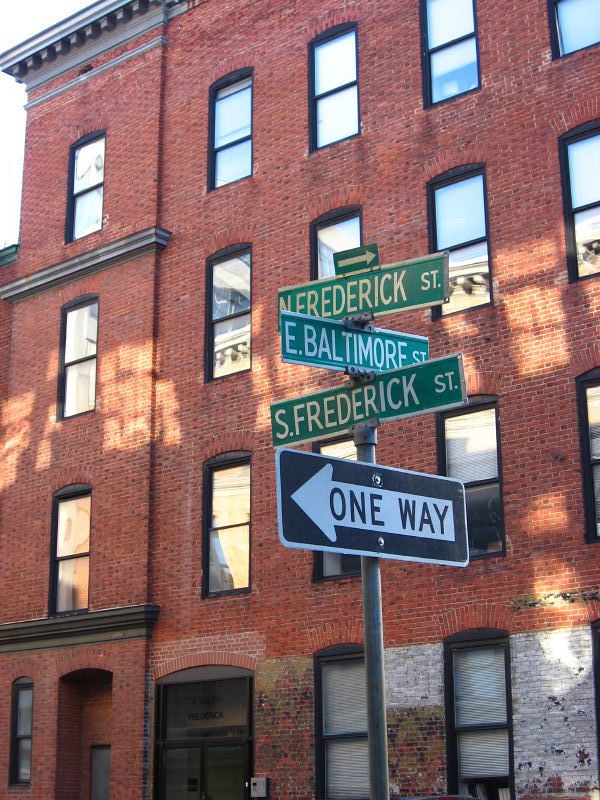The image showcases an intricate arrangement of street signs in an urban setting. Dominating the foreground, a black "One Way" sign points left. Directly intersecting this sign are two others: one indicating "South Frederick Street" heading leftward in the image, and another indicating "North Frederick Street" heading rightward. Running parallel to the "One Way" sign is an "East Baltimore Street" sign. The background reveals a charming, old red-brick building, estimated to have four stories, adorned with windows at regular intervals. At the building's base, a touch of white paint contrasts with the predominantly red brick façade, adding a layer of historical character to the scene.